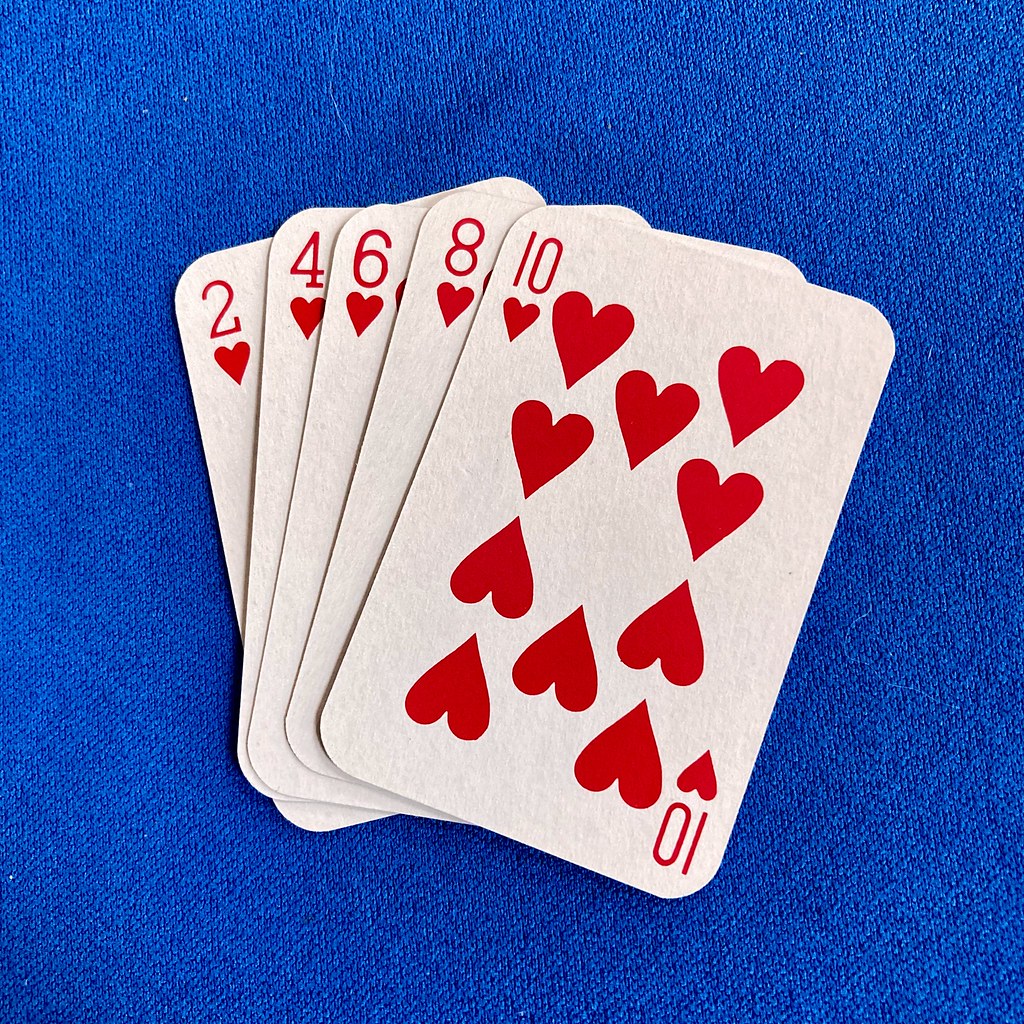This photograph features a vibrant, ultramarine blue fabric background, possibly a tablecloth. The fabric is characterized by a single white hair near the center-left edge. On top of this background, there are five playing cards, neatly stacked with only the top left corner of each card visible, except for the top card which is fully displayed. 

The cards, all with rounded edges, reveal the following sequence from the bottom to the top: Two of Hearts, Four of Hearts, Six of Hearts, Eight of Hearts, and the fully visible Ten of Hearts. The Ten of Hearts displays the number "10" and a heart symbol in both the top left and bottom right corners, along with ten heart symbols arranged in the center of the card.